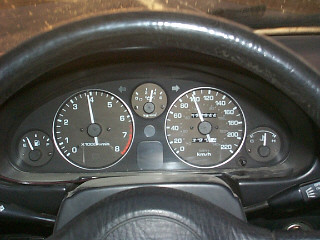This photograph offers a detailed view of an older car’s dashboard. Dominating the foreground is a thick, shiny black steering wheel that appears to be padded and covered in leather. The leather-wrapped wheel shows a hint of wear, indicating it has been well-used over time. Behind the steering wheel, a cluster of classic circular gauges is clearly visible, reinforcing the car's vintage appeal. These include an RPM gauge and a speedometer prominently displayed in the center, flanked on either side by smaller gauges for fuel level and battery status.

The base of the steering wheel seamlessly connects to the steering column, extending toward the dashboard where the gauges reside. At the very top of the image, slightly blurred, is the car’s windshield, adding a sense of depth to the photograph. To the right, a small portion of the dashboard can be seen, suggesting the presence of additional controls or features, albeit only a sliver is visible. The composition effectively captures both the timeless design and the functional aspects of an older car's interior, steeped in automotive nostalgia.